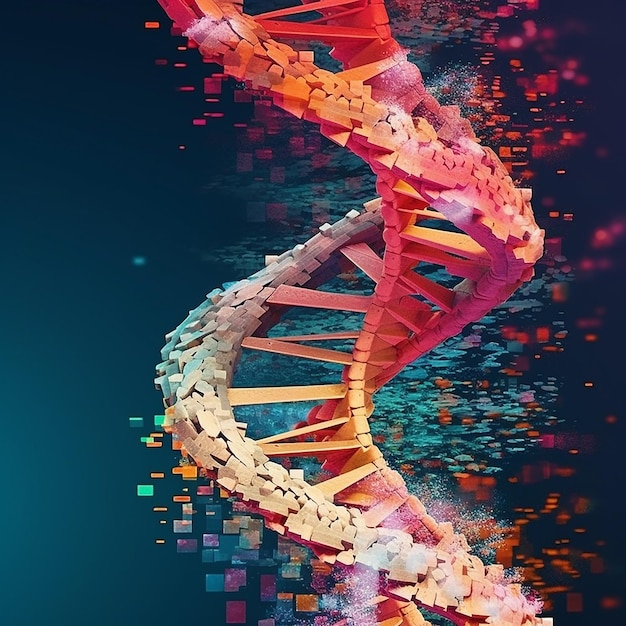The image is a graphic design resembling both a DNA double helix and a spiral staircase, set against a dark navy blue background. The helix starts from the bottom center-right and ascends, curving right then left, gradually tapering off at the top middle of the image. The helix is composed of an array of colorful squares and small shapes, predominantly turquoise, dark red, orange, yellow, green, blue, and pink. The left side features gray blocks and rocky chunks, while the right side is more colorful with a mixture of squares and circles. The strand appears like thin planks reminiscent of delicate steps in a staircase, with no railing. Adding to the dynamic visual are the surrounding splotches of blue, purple, and orange hues that pepper the background. Overall, the design is vibrant and abstract, blending both organic and structural elements seamlessly.